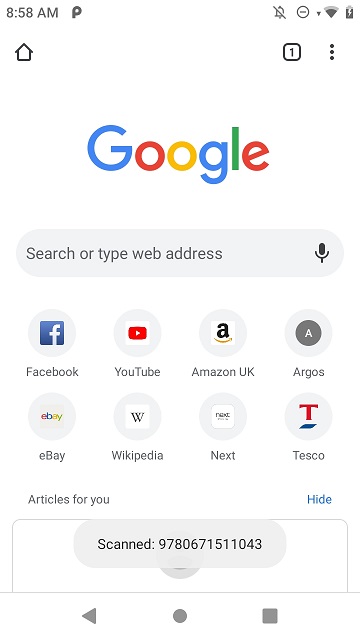This image depicts a smartphone screen displaying the Google homepage at 8:58 AM. At the top, there is a small icon of a house. To the right, there is an icon of a muted bell, followed by a circle, a triangle, and a nearly full battery symbol. Below, a black square with the number "1" inside is visible, followed by three dots. 

The word "Google" is prominently displayed in large, multicolored letters (blue, red, yellow, blue, green, and red). Beneath the Google logo is the search bar with a microphone icon on the right side.

Listed below the search bar are quick access icons for several popular websites: Facebook, YouTube, Amazon UK, Argos, Ebay, Wikipedia, Next, and Tesco. Below these icons, there is a section titled "Articles for you," with a "Hide" option in blue text to the right. 

There is also an area showing a scanned item with a long oval shape around the text "scanned" in black lettering, alongside the number "9780671511043." At the bottom of the screen, navigation icons for a back arrow, a circle, and a square are visible.